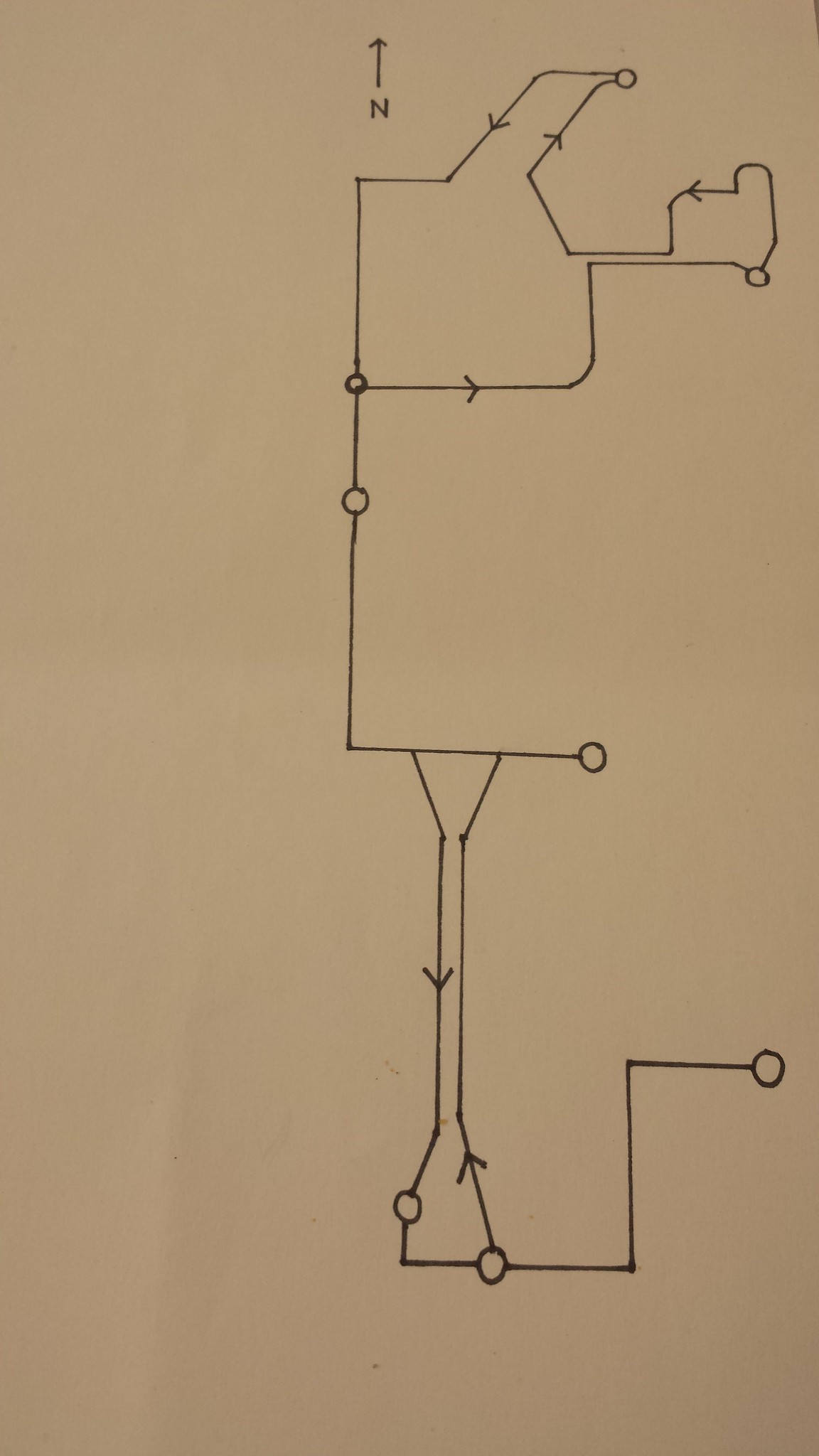**Portrait Mode Map Diagram**

The diagram, drawn in thick black marker on a light brown paper background, appears to be a map with a northward orientation indicated by an "N" with an arrow pointing upward at the top center. 

- **Bottom Right Corner:**
  - A circle is situated just above the bottom right corner.
  - A line extends leftward from this circle, then turns down, then left again to lead to another circle.

- **From the Second Circle:**
  - An arrow points upward from the top.
  - A line extends left and then upward to a third circle.
  - From this third circle, a line bends to the right, running almost parallel to the vertical arrow line.

- **Parallel Lines:**
  - One line (from the third circle) continues up with an arrow pointing down partway along.
  - The other arrow line, on the right, continues upward before branching right into a line that ends in another circle.

- **Circle and Line Intersections:**
  - The circle line on the left continues upward, meeting another line that extends left to a fourth circle.
  - From the fourth circle, a line goes left and then angles upward to a fifth circle near the center left.

- **Top Section:**
  - From the fifth circle, a line goes upward to a sixth circle, which has two branching lines:
    - One line goes right, curving up and ending in an arrow before continuing upright.
    - The other line goes straight up to a seventh circle. From this seventh circle:

- **Complex Path at Top Right:**
  - A line extends up, then curves right, and continues straight upright.
  - It then bends down, continuing left to become parallel with a previous horizontal line.
  - This line then curves left again, leading to an eighth circle near the top right-center of the diagram.

- **Final Connections:**
  - From the eighth circle, a line bends left, curves down with an arrow marking the direction.
  - This line ultimately curves back leftward, meeting another flat line.
  - The diagram ends in a downward line that reconnects with the sixth circle.

The diagram's intricate network of lines, arrows, and circles may indicate a detailed schematic or pathway of some kind, which could potentially represent a map or flowchart.